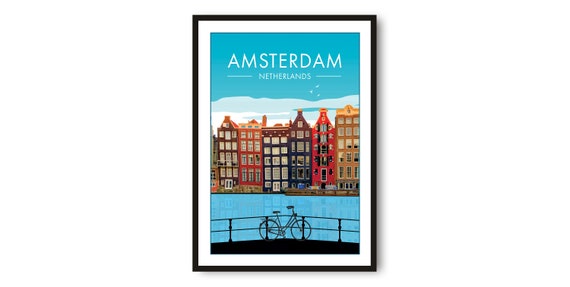This photograph features a vibrant, framed poster of Amsterdam, set against a white mat within a sleek black frame. Dominating the top of the poster, bold white block letters spell out "Amsterdam" against a cyan sky dotted with white clouds. Below, centered in smaller white block letters, is "Netherlands," flanked by two narrow white lines.

The scene transitions into a bustling cityscape characterized by tall, narrow buildings reminiscent of Amsterdam’s iconic architecture. The multi-story buildings vary in color, including shades of maroon, red, brown, yellow, and beige. Each structure is interspersed with numerous windows, distinctly outlining their silhouettes.

Beneath this urban skyline flows a broad, tranquil canal depicted in a vivid sky-blue hue. In the foreground, a sturdy metal railing with two round rails, subtly frames the view. Parked against this railing is a bicycle, providing a quintessentially Dutch touch to the tableau. A dark, black path anchors the foreground, completing the picturesque scene of the city.

This simple yet evocative image captures the essence of Amsterdam, showcasing its unique blend of architectural charm and serene waterways.